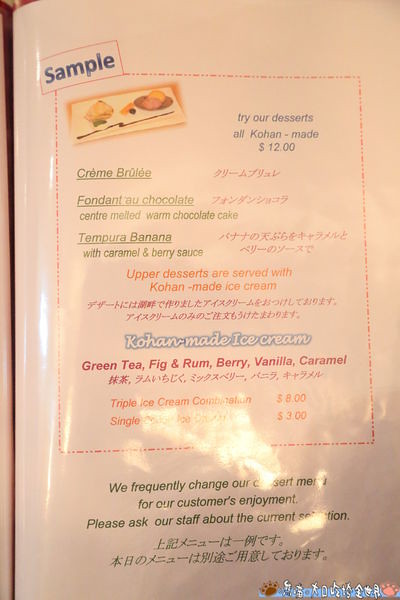This image displays a page from a menu titled "Sample." At the top, an icon depicting indistinct food items is shown. The menu lists several desserts, all crafted in a Cajun style, priced at $12. The offerings include crème brûlée, fondant au chocolat featuring a warm melted chocolate center, and tempura banana with caramel and berry sauce. These desserts are noted to be served with Cajun-made ice cream. The ice cream flavors listed are green tea, fig and rum, berry, vanilla, and caramel, with a triple ice cream combination priced at $8 and a single scoop at $3. Additionally, there is a note stating that the menu frequently changes for customer enjoyment, prompting patrons to ask the staff about the current selection. The menu also features writing in an Asian language, adding to its diverse presentation. The background of the menu is pink, and there's a small sunshine icon along with a photograph of candy and ice cream at the top. Near the bottom, part of the text is obscured by a bright reflection.